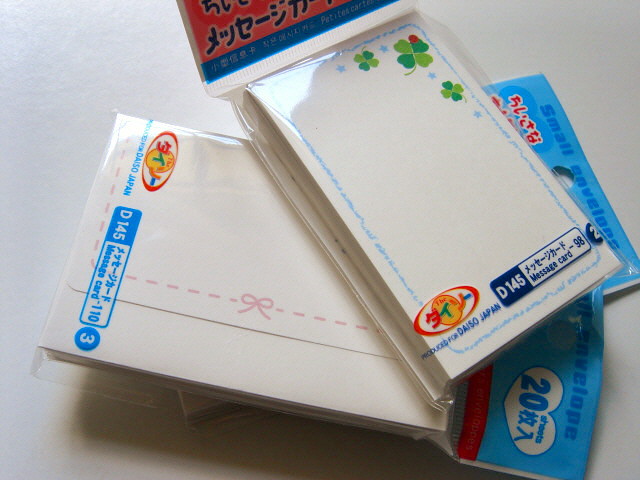The photograph depicts two packages of notepads displayed against a white background, resembling a tabletop. Each notepad is wrapped in clear plastic and topped with a blue and green label displaying Asian characters, likely Japanese. The packages are designed for store display, featuring a hole for hanging on a rack. Visible are two primary notepads: the top one is white with a blue border and adorned with three four-leaf clovers—two light green and one dark green—alongside four small blue stars. The second notepad is white with a pink segmented line running vertically and a pink bow at the bottom. Both packages prominently feature the detailed and simple designs, aimed at being visually appealing while maintaining functionality.